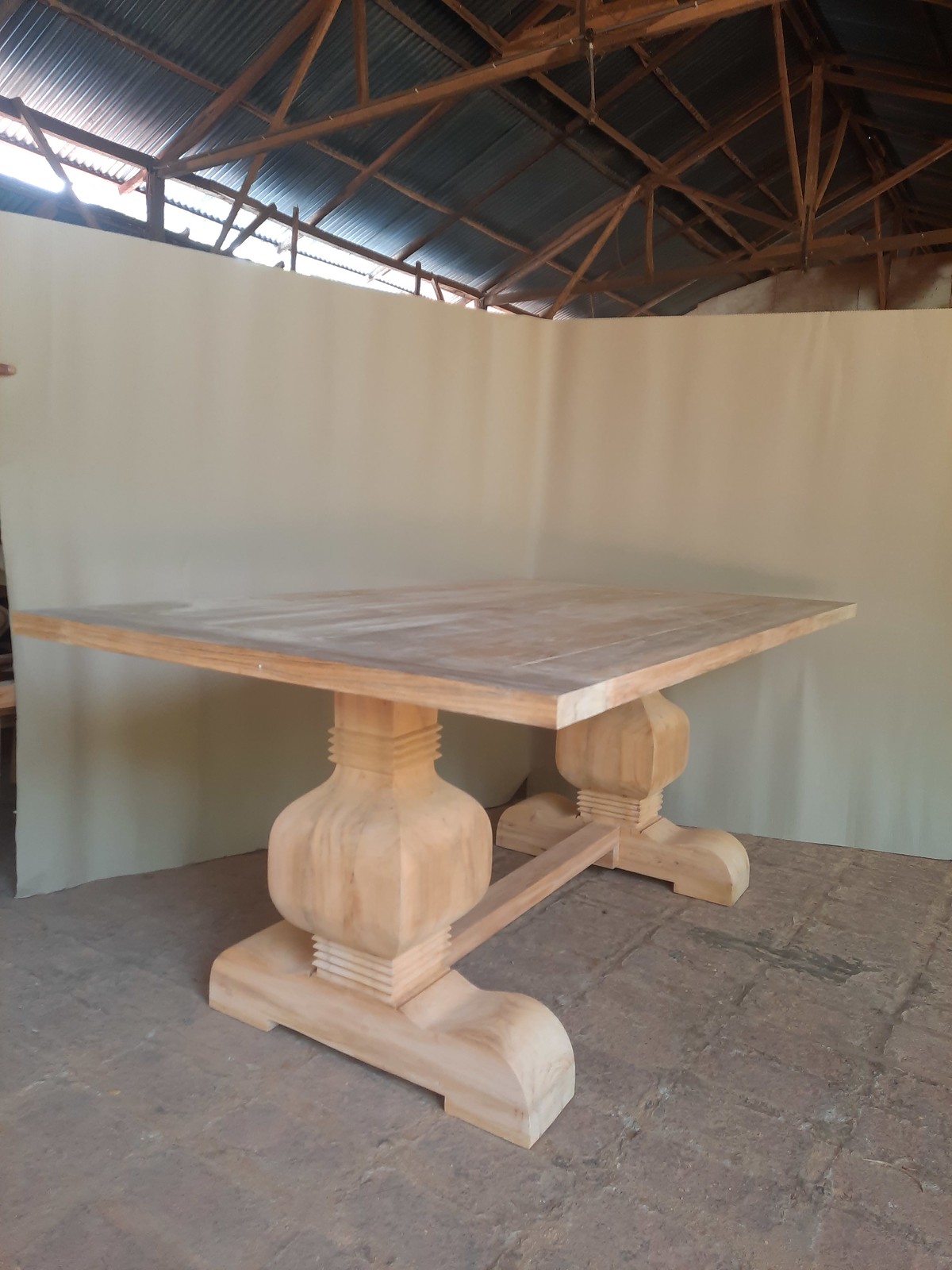The image depicts a handcrafted light brown wooden table with a layer of white dust on its surface. The table stands on a concrete brick floor, featuring two pedestal legs that widen into somewhat cube shapes mid-leg, connected by a beam at the bottom for stability. Each pedestal leg has wide, large feet extending from its base. The setting appears to be a storage or pole barn under construction, with metal rafters supporting a tin roof above. There is a simple white curtain along the back of the table, sectioning off the area, which is illuminated by light filtering through the rafters. The space, albeit dusty and unfinished, adds to the rustic charm of the wooden table.